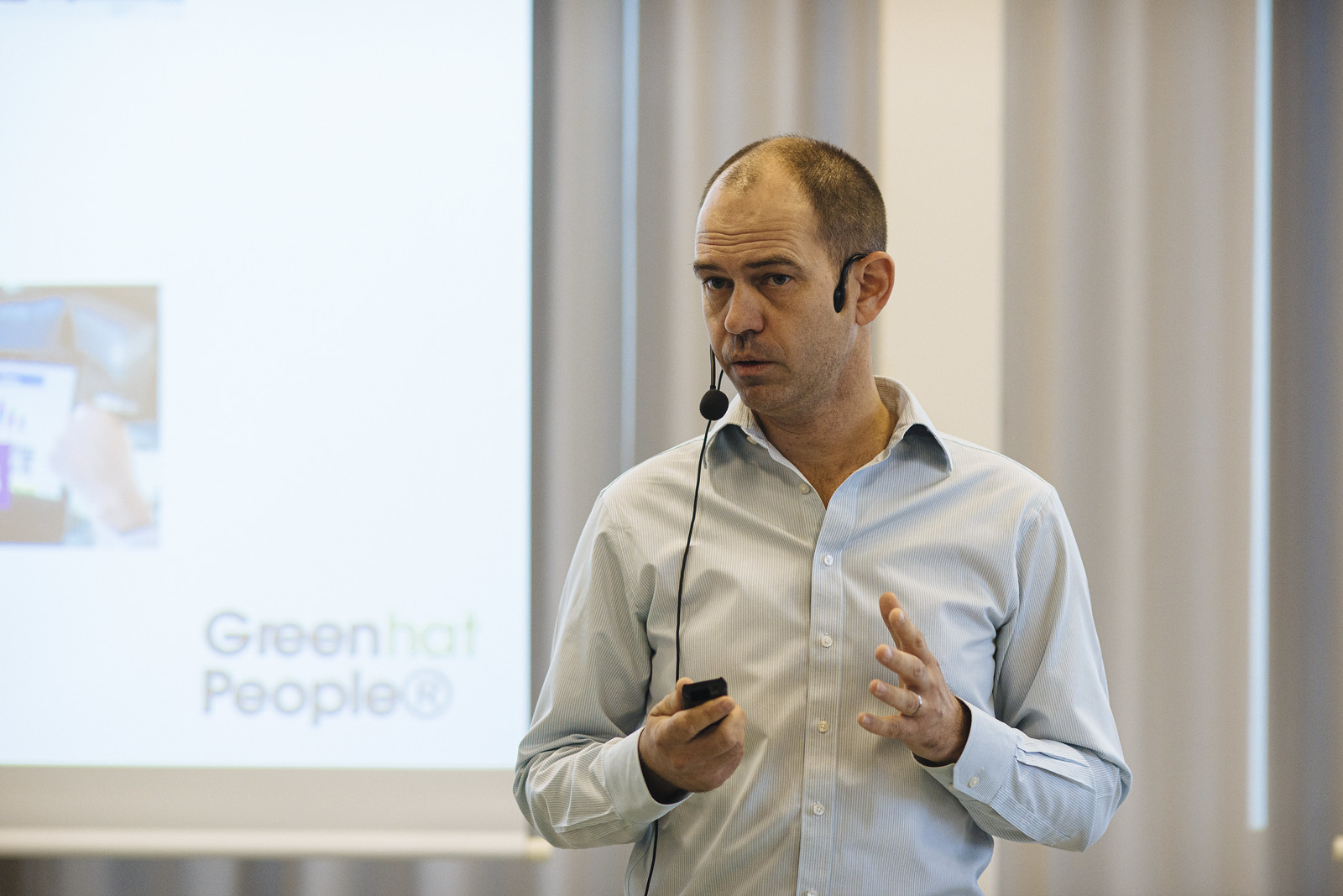In this image, a man, presumably giving a lecture or presentation, stands centrally within an indoor workplace setting. He is clothed in a light blue, slightly unbuttoned, long-sleeve button-down shirt. The man is wearing a headset with a microphone positioned in front of his face. His left hand, adorned with a ring, is extended outward as if gesturing during his speech, while his right hand holds a black remote or clicker. The man has balding brown hair and no tie.

Behind him, the backdrop consists of white, light brown, and blue curtains, with light filtering through them, possibly from a window covered by blinds. To the left side of the image, there is a pull-down projector screen displaying the text "Green Hat People" in blue letters, along with an indistinct, blurry picture that appears to depict a computer monitor or a laptop with an image resembling Earth and outer space. The setup suggests a professional or educational environment, underscored by the man’s poised, speaker-like demeanor.